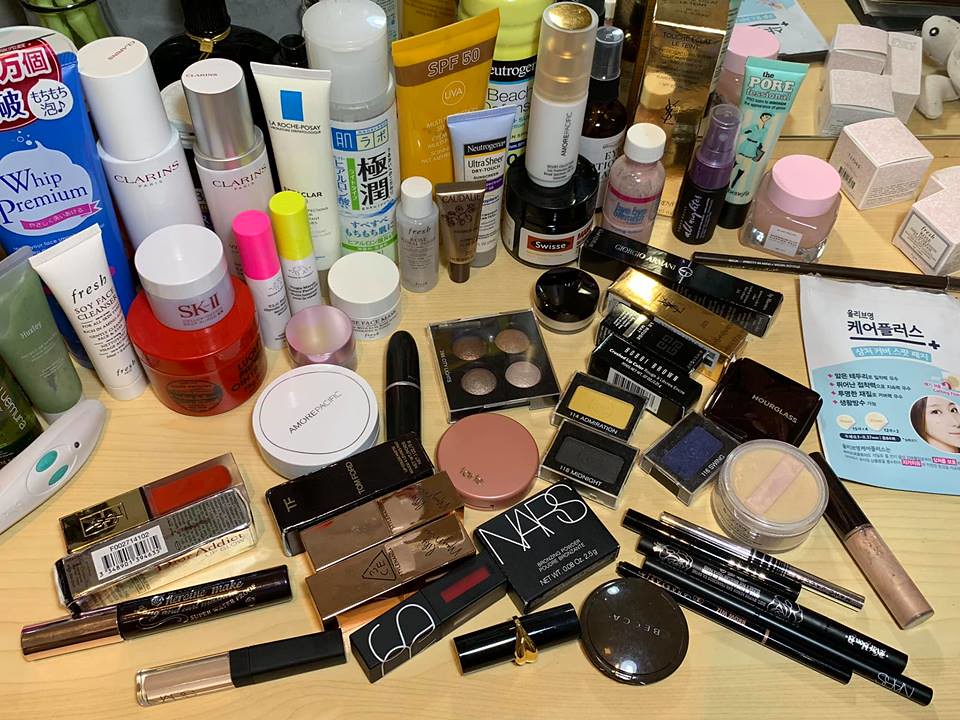A neatly organized vanity is filled with a diverse assortment of high-end makeup and skincare products. In the front, prominently displayed are a variety of makeup items from renowned brands such as NARS, Bobbi Brown, Hourglass, and Armani. You can spot blush, eyeshadow, lipstick, mascara, and eyeliner among these. Towards the back, there is an array of skincare products including setting sprays, sunscreens, moisturizers, and cleansers. Notably, there is a Neutrogena sunscreen positioned towards the front. A sheet mask with writing in an Asian language, potentially Chinese, is also visible, hinting at the owner's interest in international skincare products. The overall appearance suggests that these products are relatively new and well-maintained, showcasing someone's carefully curated beauty collection.